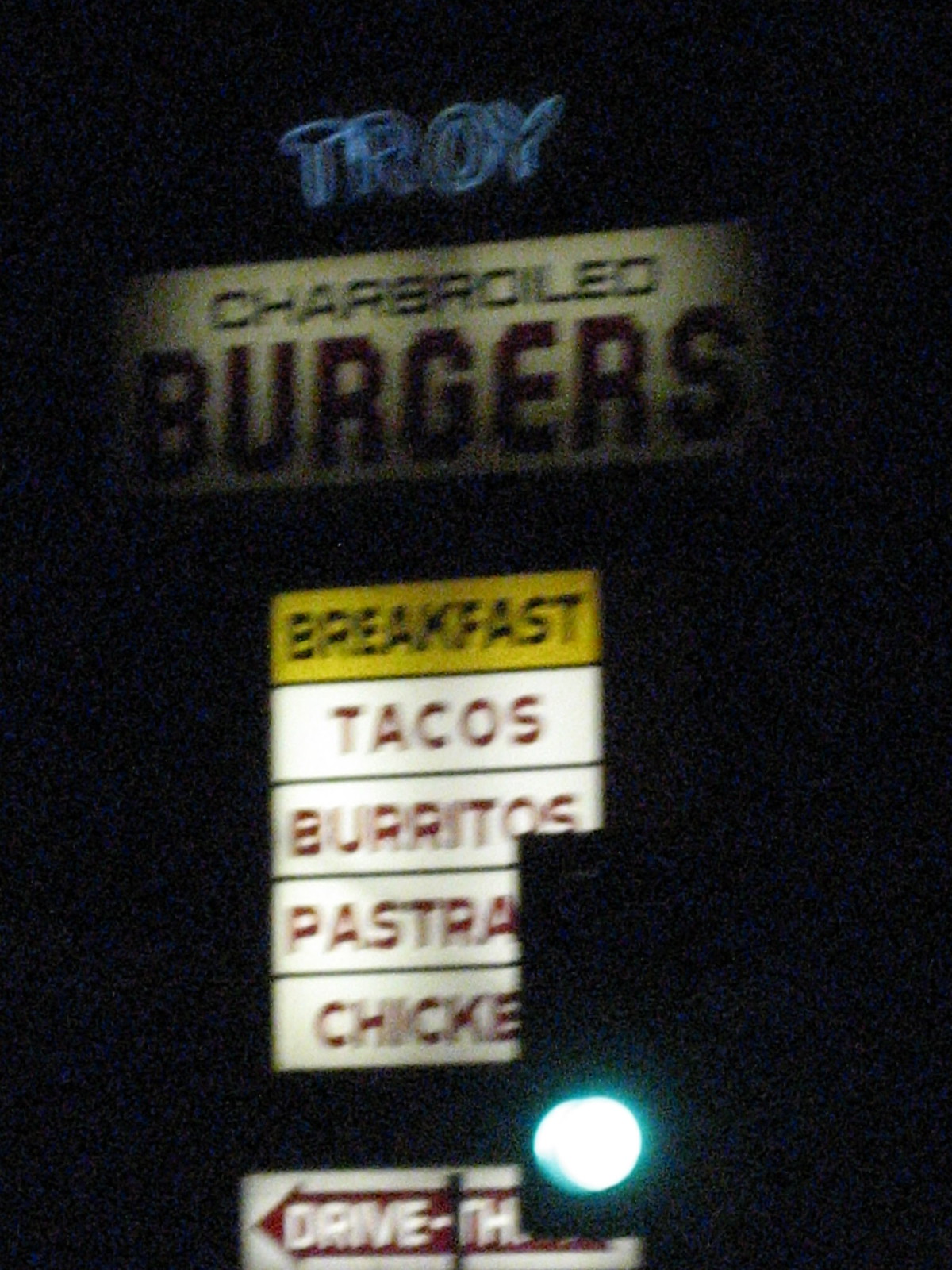This nighttime scene features a vividly illuminated restaurant sign. The primary sign reads "Troy" in a striking bright blue outline, adding a modern touch to the dark surroundings. Directly beneath this, another glowing sign displays "Charbroiled Burgers" in bold lettering. The word "Charbroiled" appears in black, while "Burgers" is rendered in red, creating a clear and appetizing highlight.

Further below, a yellow sign with black text announces "Breakfast," while another sign lists menu items: "Tacos," "Burritos," "Pastrami," and "Chicken," all presented on a white background with red lettering. Beneath these, yet another sign points to a drive-thru to the left, with a red arrow and text that matches the motif. The arrow and its interior letters are brightly illuminated in red and white, ensuring night visibility.

To the right of these signs, a traffic light shines green but partially obstructs the view. It covers the "N" in "Chicken" and partially obscures some letters in "Pastrami" and "Burritos." This collection of vibrant colors and lights against the night sky makes the restaurant's presence boldly known.